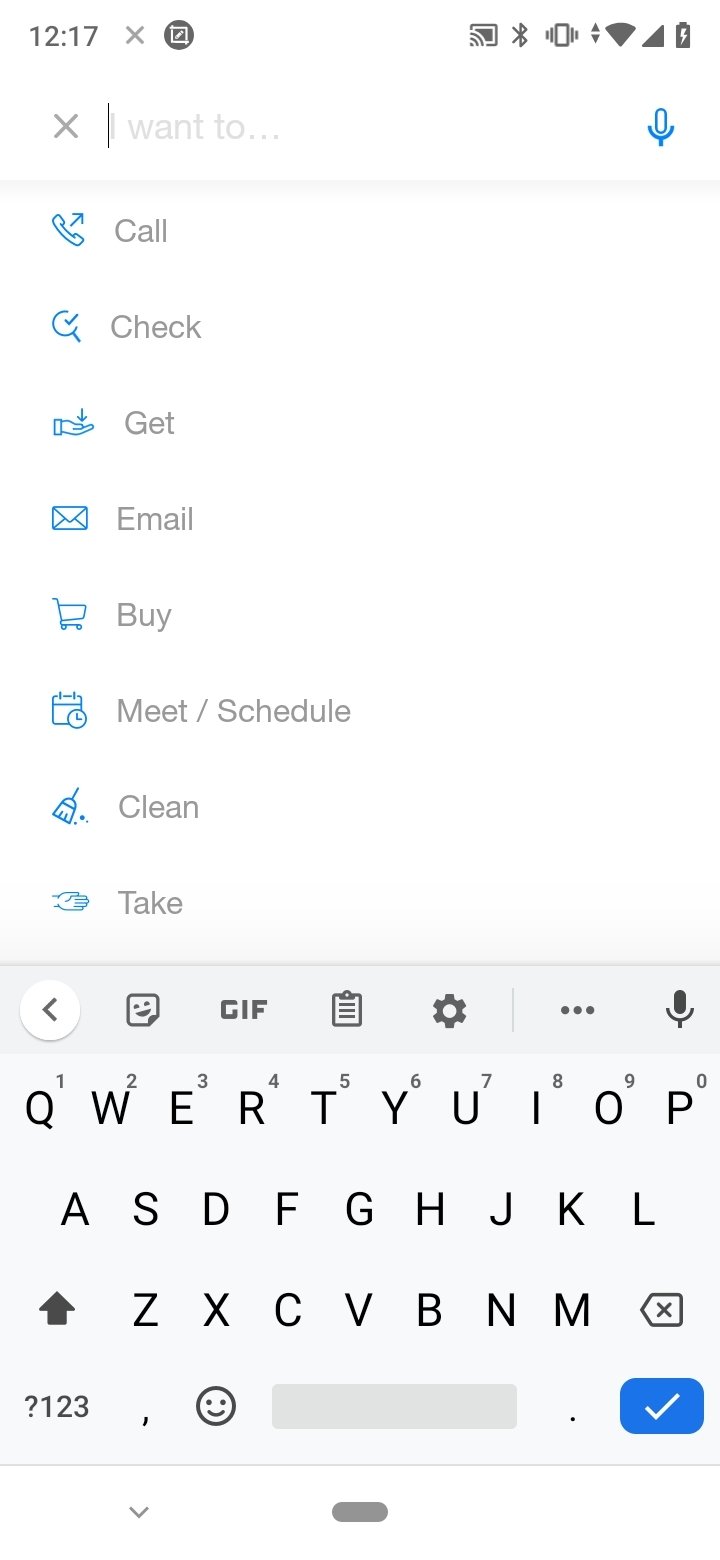The image displays a smartphone screen showcasing a productivity app. The current time on the phone is 12:17, as indicated by the status bar, which also shows icons for casting, Bluetooth, haptics, full Wi-Fi, full signal strength, and a fully charged battery. 

The main interface of the app features a text field labeled "I want to," with a blinking cursor ready for input. To the right of the text field, there's a light blue microphone icon, suggesting voice input capability. Below this, a series of blue icon-labeled options are listed, including 'Call,' 'Check,' 'Get,' 'Email,' 'Buy,' 'Meet,' 'Schedule,' 'Clean,' and 'Take.'

A QWERTY keyboard is visible at the bottom of the screen, overlaying the app's interface. The keyboard includes buttons for adding GIFs, attachments, and voice typing, as well as a gear icon for accessing settings. The keys have a black background, contrasting with the white background of the app. 

In the lower right corner of the screen, there's a prominent blue button with a white checkmark. The overall layout and numerous options suggest that this app is designed to help users manage various tasks efficiently.